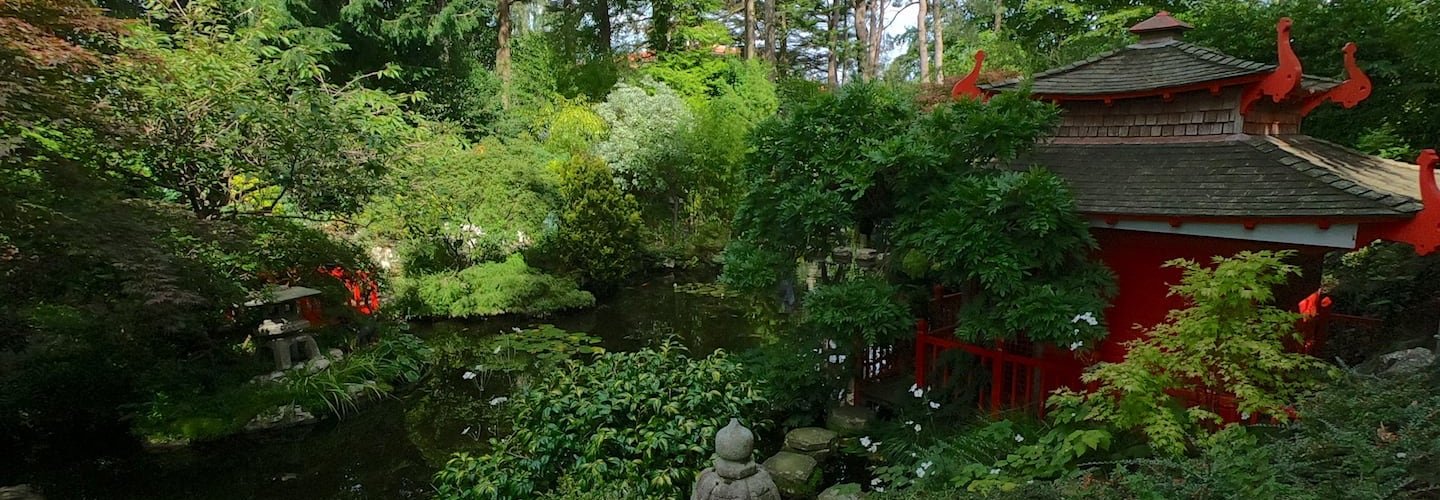The outdoor photo showcases a lush, vibrant garden that evokes a sense of serene beauty, possibly reminiscent of Japanese or Chinese landscapes. The scene is dominated by an abundance of green plants, tall trees, and flourishing shrubbery. A small pond or creek snakes through the center, surrounded by various flowers in shades of pink, purple, and red. 

Toward the lower section of the image, a small gray statue adds a nuanced touch of tranquility. Standing on the right side is a striking red structure with a traditional, tiled roof featuring decorative hooks or dragon-like ornaments at each corner, adding an architectural allure. The roof is composed of two layers, with the main layer supporting a smaller, elevated section. 

In the distant left side, another small statue can be seen, complementing the scenery, while colorful red flowers peek through the foliage. Behind this vivid tapestry of greenery and blossoms, tree trunks rise up against a backdrop of clear blue sky, completing the enchanting landscape. The image encapsulates a picturesque, well-tended garden brimming with natural beauty and intricate details.